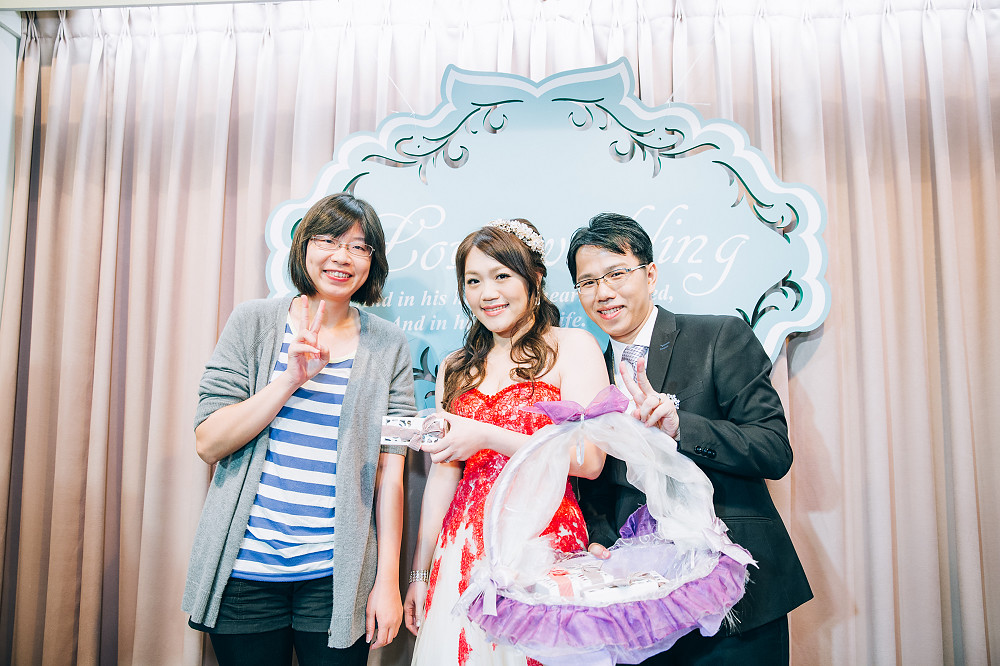The photograph shows three people of Asian descent, all smiling and posing for the camera with victory symbols made with their fingers. The woman in the center, with long auburn-brown hair styled in a floral bun, wears a low-cut red formal dress that leaves her shoulders bare. She is holding a rectangular award or prize decorated with ribbons and bows. The woman on the left has short dark hair and glasses, and is dressed in a grey cardigan over a blue and white striped top, with shorts over tights. The man on the right, who has black hair and glasses, is wearing a dark suit coat with a necktie. Behind them, a light blue sign with white font is partially blocked by their poses, and beige curtains are visible in the background.